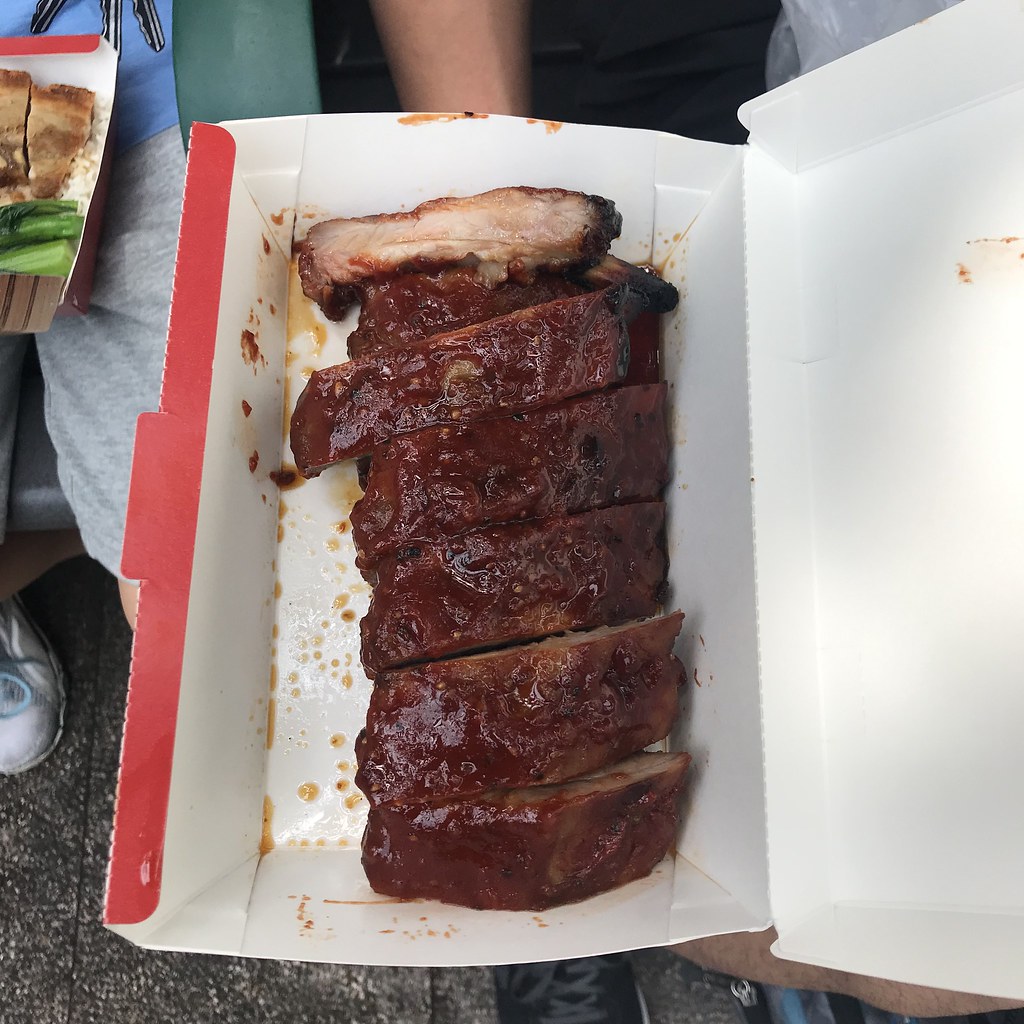The photograph captures a takeout tray filled with what appears to be barbecued short ribs. The brown meat, cut into long, narrow sections, is generously smothered in a thick red barbecue sauce, with some sauce and grease pooling in the tray. The primarily white interior contrasts with the red exterior of the box. A hand, barely visible in the bottom right of the image, holds the tray up to the camera. The person holding the tray is wearing gray sweatpants, a blue t-shirt, and possibly a green vest. In the top left of the image, there's another similar takeout box on the person’s lap, containing chunks of golden meat, green vegetables, and what looks like a bed of white rice.